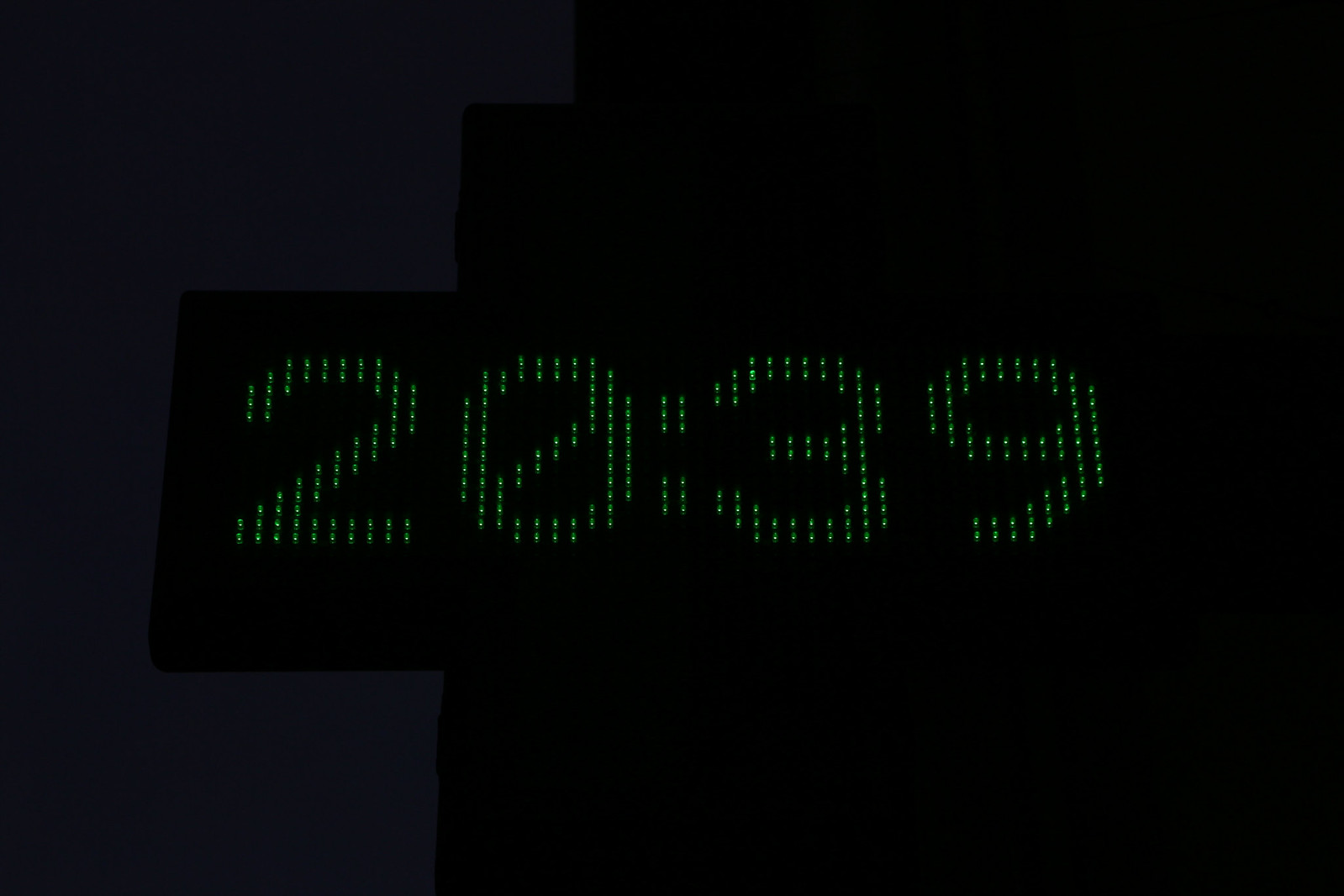The image showcases a digital clock against a predominantly black background. The clock displays the time as "2039", formed by small, illuminated green dots. Each number is composed of these tiny lights, creating a bold and striking appearance. The green digits are large and centrally positioned on what appears to be a dark building with jagged, geometric edges. To the left of the image, the black background fades into a very dark blue, reminiscent of a night sky. The futuristic style is emphasized by the precise arrangement of the lights, with each line of the numbers being roughly two dots wide and a slight halo effect encircling the brighter centers. Notably, the zero digit features a diagonal line running from its bottom left to top right.